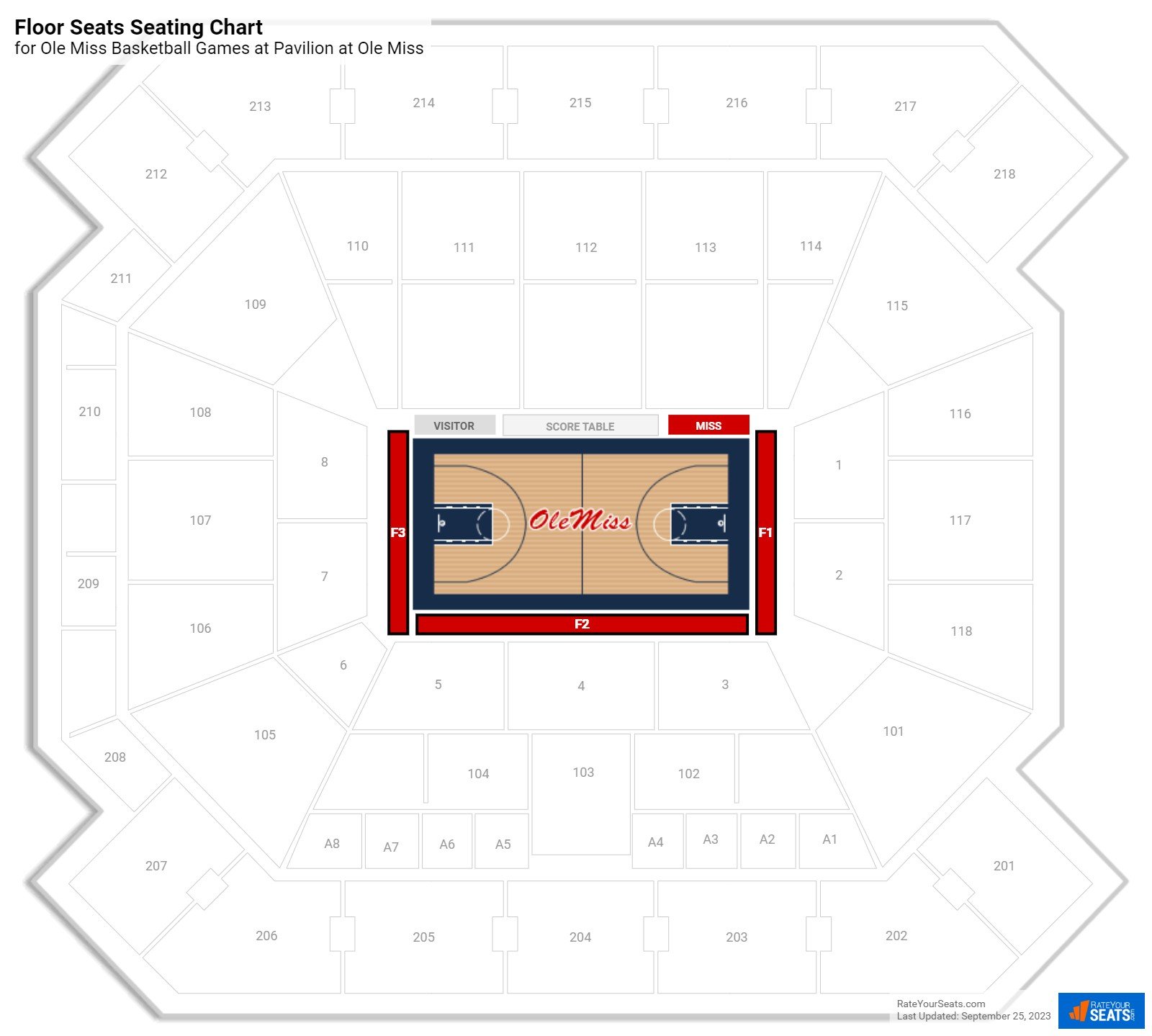This image is a detailed screenshot from a website, providing an overhead view of a stadium's seating arrangement centered around a basketball court marked "Ole Miss." The court itself is framed by a navy blue border and clearly visible sidelines. The right sideline is labeled "F1," the bottom sideline "F2," and the left sideline "F3." At the top of the court, sections are marked as "visitor," "score table," and "miss," all highlighted with a red background.

Surrounding the court, the seats are sequentially numbered. Directly behind the F1 section, seating sections 1 and 2 are visible. Adjacent to F2, sections 3, 4, and 5 are labeled, while the area behind F3 includes sections 7 and 8. A corner area, marked as section 6, connects these seating arrangements. There is a noticeable gap with no seating immediately behind the "visitor," "score table," and "miss" sections, which resumes at the second row at the top. Seating numbers continue to increase, reaching up to 218 in the topmost corner, providing a comprehensive layout of the stadium's seating arrangement.